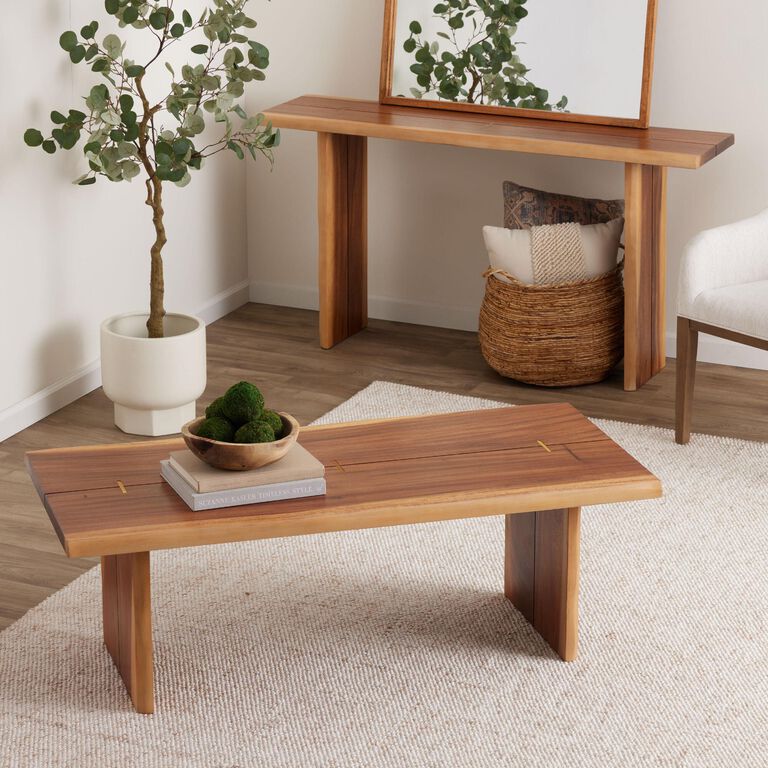The image depicts a cozy corner, likely of a living room, featuring a brown, wooden laminate floor complemented with a tan, beige rug. Positioned centrally is a wooden stool table, which holds two books— the bottom one light blue and the one on top tan-colored— along with a bowl that has green elements, possibly decorative balls. In the background, the white walls are accented by a white pot housing a tree with a mix of dark green and light green leaves. To the right edge, a glimpse of a white chair is visible, indicating a seating area. On one side of the wall, there's a tall, skinny table, possibly with a mirror on it, and below it, a basket filled with pillows.